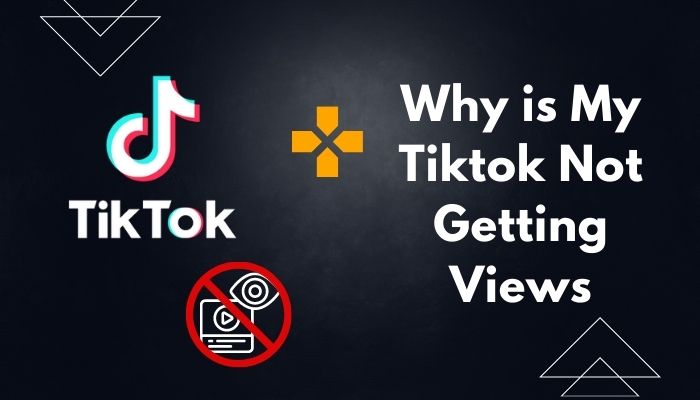In this advertisement for TikTok, the central feature is the prominent TikTok logo, which consists of a white musical note and the text "TikTok" with both the T's in "Tik" and "Tok" capitalized. To the right of the logo, there is an orange circle with an "X" in the middle, followed by the text "Why is my TikTok not getting views?" in white. 

Above the TikTok logo, there is a graphic displaying a pair of double triangles with their pointed ends facing down, mirrored by a similar set of triangles in the bottom right corner pointing upwards. Below the TikTok logo and slightly indented to the right, there is an icon resembling a video play button with a red crossed-out eye symbol overlaying it, indicating "no views." 

The entire advertisement is set against a black background with white text. The design features a subtle gradient effect where the edges are a darker black, gradually lightening to a faded white towards the center, creating a spherical highlight effect. This enhances the focus on the central elements of the ad.